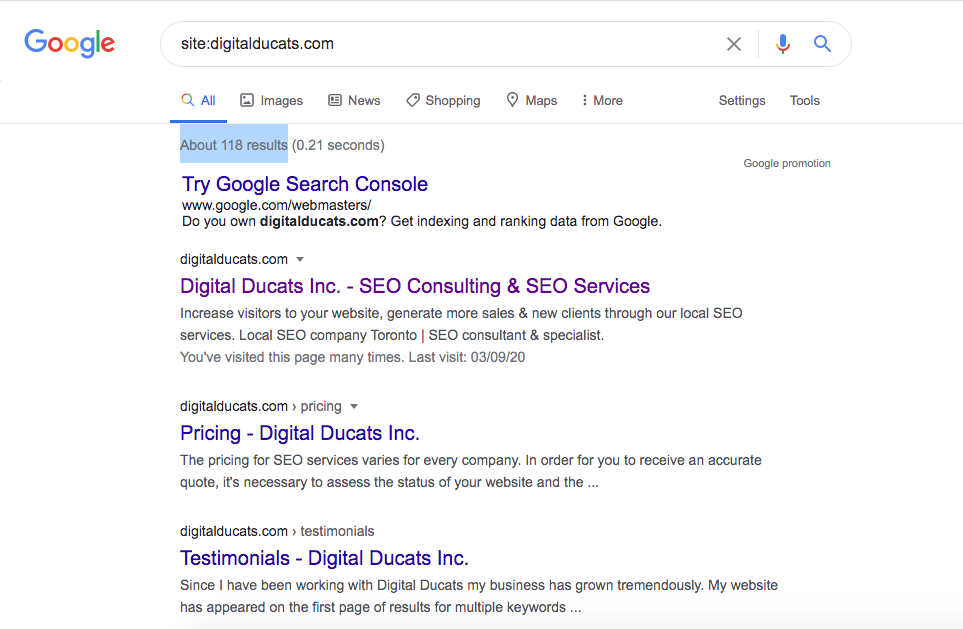In this image set against a solid white background, the upper left corner features the iconic Google logo in its standard colors of blue, red, yellow, and green. Positioned to the right of the logo is a search bar containing the text "site:digitalduckcats.com" in black. Below the search bar, the first search result stands out with text highlighted in blue, which reads: "Try Google Search Console - www.google.com/webmasters.” The snippet beneath the title addresses the viewer directly with, "Do you own digitalduckcats.com? Get indexing and ranking data from Google." The detailed description for the search result includes a promotional message for DigitalDuckCats.com, advising to "increase visitors to your website, generate more sales and new clients through our local SEO services. Local SEO Company Toronto, SEO Consultant and Specialist." A notation indicates that the viewer has visited this page many times.